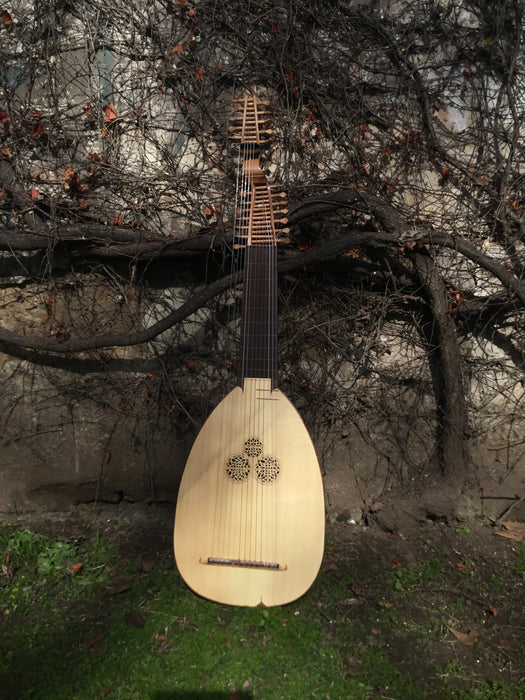The image features an outdoor scene with a vintage, birch or light brown maple wood lute prominently displayed in the foreground, leaning against the dark, bare branches of a low-lying tree. The instrument's pear-shaped body showcases three sound holes arranged in a triangular fashion. The dark brown and black fretboard features multiple layers of strings, possibly up to 12, and an elaborate bridge. In the background, there are additional trees with sparse foliage, revealing a light, airy backdrop through the branches. The ground is a mix of black dirt, rocks, and patches of green grass, adding to the rustic and natural aesthetic of the scene. It almost seems like there might be another similar instrument partially hidden behind, adding to the layered, textured composition of the image.